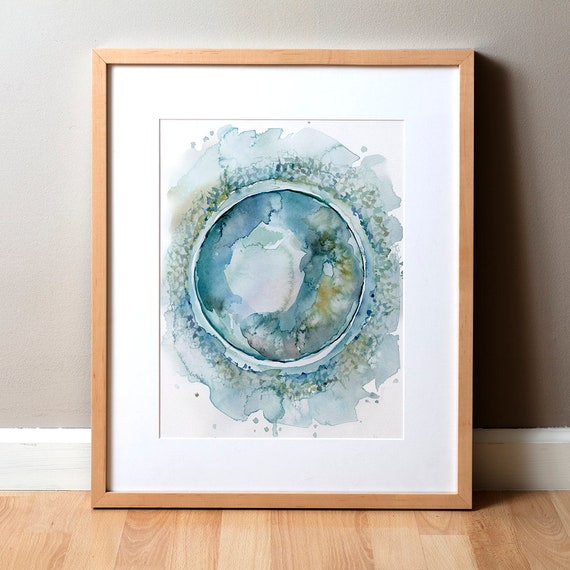The painting is displayed in a thin tan wooden frame, with a thicker white border surrounding the artwork itself. The watercolor painting, which evokes an abstract representation of the Earth or an eye, features a central circle in blue and green shades, surrounded by petal-like blobs and irregular strokes that extend outward. The colors in these outer regions include blues, greens, yellows, and some areas of dotting and speckling, creating a dynamic and textured appearance. The painting, which sits on a light brown wooden floor, rests against a tan-colored wall with a white crown molding at the bottom. Shadows are cast against the grey-toned wall, adding depth to the scene.